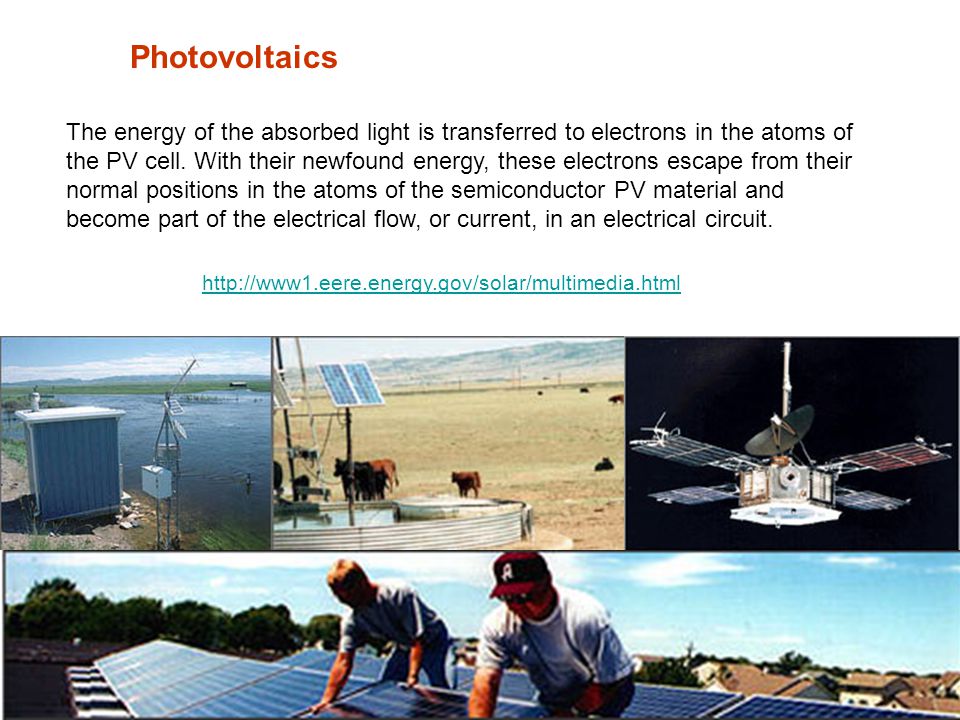The image features an informative paragraph at the top with the title "Photovoltaics". The description explains that the energy from absorbed light is transferred to electrons in the atoms of a photovoltaic (PV) cell. With their newfound energy, these electrons escape their normal positions in the atoms of the semiconductor PV material and become part of the electrical flow or current in an electrical circuit. Below this text is a light green URL link to http://www1.eere.energy.gov/solar/multimedia.html. 

Arranged below in two rows, the image showcases four photographs. The first row consists of three smaller images: the left shows a white shed with a blue front next to an antenna and a body of water under a blue sky; the middle image features solar panels with several cows grazing in a brown field with mountains in the background; and the rightmost image depicts a satellite suspended against a dark background. The lower, elongated rectangular image shows two men installing solar panels on a house roof, with rooftops of other houses and a blue sky with white feathery clouds visible in the background. One of the men, wearing a red baseball cap with the letter 'A' in white, is seen alongside his colleague in short-sleeved shirts and jeans.